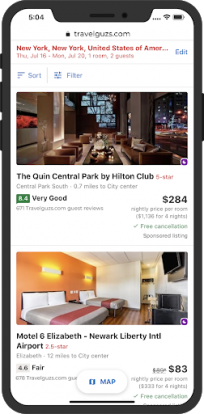The image features an iPhone screen displaying a webpage from travelguz.com. The current time shown at the top of the screen is 5:04, and the phone's battery is nearly full. The website appears somewhat blurry but reveals a travel quiz with various details prominently highlighted.

At the top of the webpage, text in red states: "New York, New York, unlimited state, United States of America." The date is given as Thursday, July 16th. An edit button in blue is positioned on the right side of the screen.

The page showcases a visually appealing image of a hotel interior identified as "The Quin Central Park by Hilton Club," rated five stars in red. It is described as "very good" and priced at $284. Additional information is provided in fine print in black, including a green check mark indicating "free cancellation."

Underneath this section is another listing with an image labeled "Motel 6 Elizabeth Newark Liberty International Airport." This accommodation has a two-and-a-half-star rating, costs $83, and is described as "fair." 

At the bottom of the screen, there is a blue map feature that users can click on to view the locations of the listed hotels.